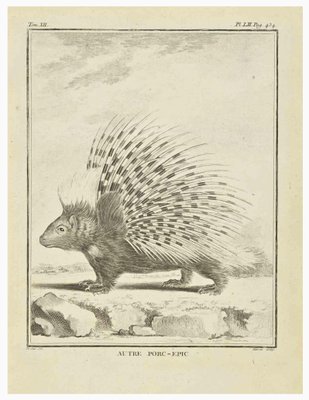This image features a detailed, hand-drawn illustration of a porcupine, extracted from an old book page with a beige, tan background. The page itself is rectangular, roughly an inch and a half wide by two inches tall, framed by a thin, light gray border. The central picture is further delineated by a thin black border. The porcupine, a rodent-like creature, is depicted standing on all fours on a stone or gravel path against a clear background, with some large rocks visible to its side. Facing left, the porcupine showcases its side profile, adorned with numerous large quills that extend outward from its back, exhibiting an alternating pattern of black and white. In the upper corners of the image, there is blurred text, while at the bottom, the text "Metroporc Epic" is somewhat more legible, identifying the creature and providing context to the illustration, giving the impression of an old, meticulously detailed, and somewhat worn page from an informative animal guide.